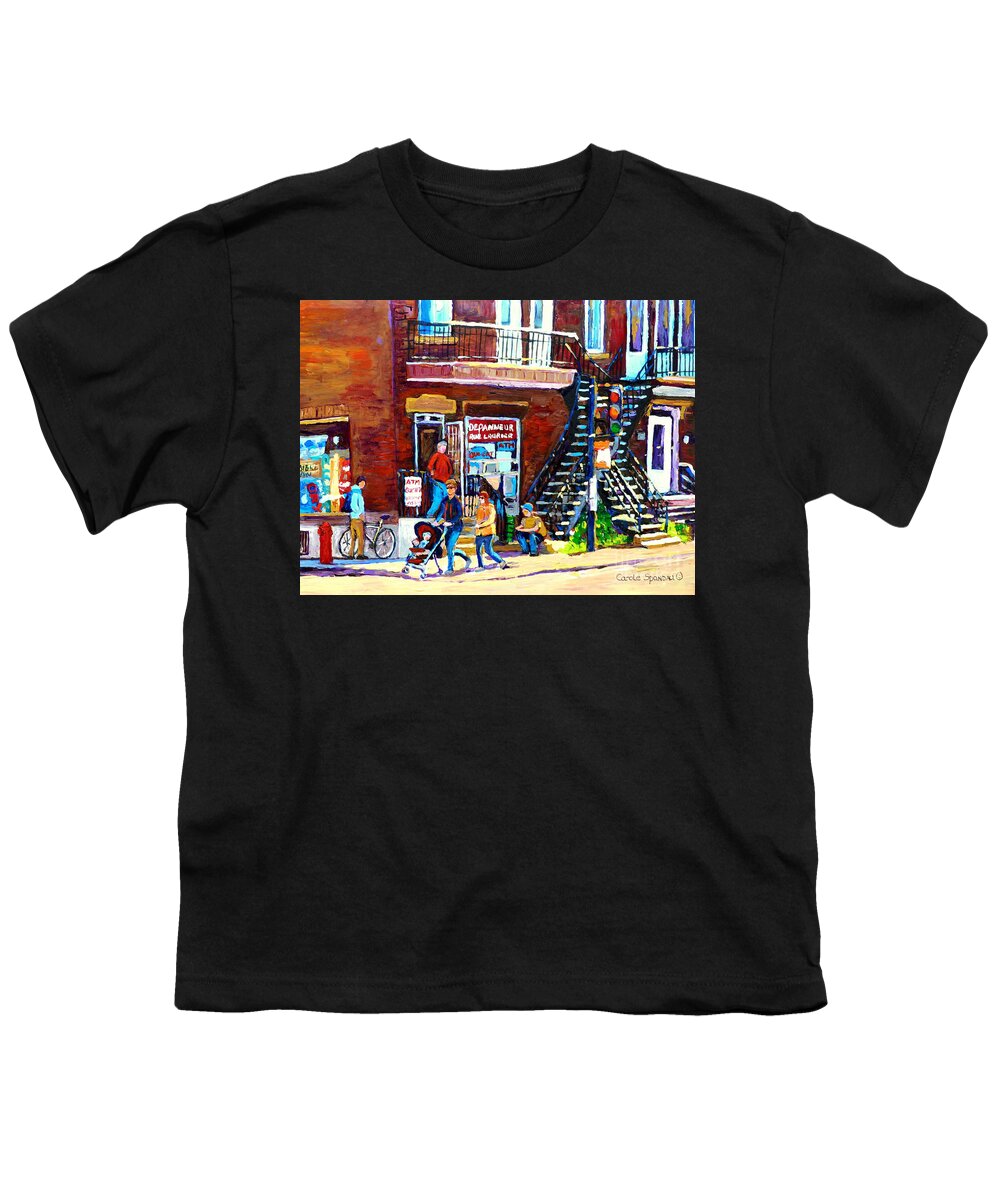This detailed image displays a black t-shirt laying flat against a plain, invisible or white background. The t-shirt features short sleeves and a black ring around the crew neck collar. Screen printed on the t-shirt is a vibrant, impressionistic cityscape artwork, titled "Rue Laurier de Pinot," which is a market scene set in Montreal. 

In the middle of the t-shirt, the artwork showcases a bustling street corner. On the left side, a brick building houses a small grocery store, identified by its glass windows and doorway, situated beneath black iron stairs that lead up to apartments above. The foreground of the image captures a dynamic street scene: 

- A man in a teal blue jacket and brown pants stands next to a bicycle propped against the grocery store wall.
- To the right, a couple, the woman in an orange coat and the man in a blue jacket, push a red and blue stroller with their child inside.
- A person sits on the bottom step of the building's steep stairs, and another person is seen exiting the corner store.

Details also include a red fire hydrant on the sidewalk and a classic stoplight with red, yellow, and green lights. The scene is framed by a beige roadway, brick buildings, and upper-story balconies, giving a true-to-life urban atmosphere. The artist's signature, “Carol Spundo :)” can be found in the bottom right corner of the artwork.